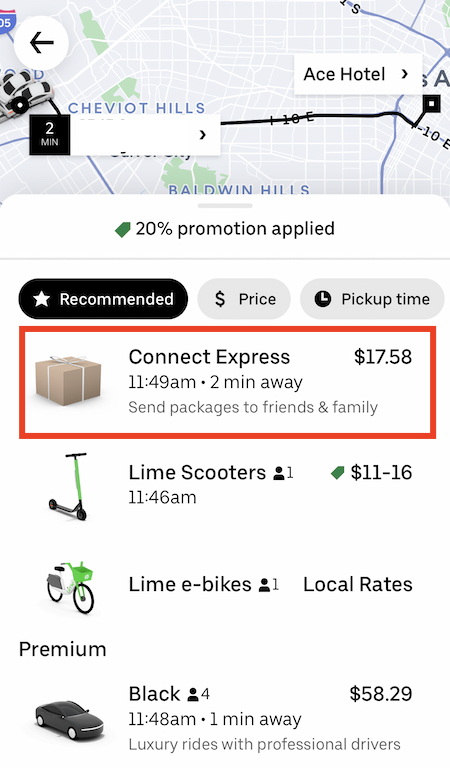A detailed caption for the given screenshot:

The image is a detailed screenshot of an Uber app interface. At the top section of the screenshot, a map is visible with a location marker indicating "Shepboy Hills." Additionally, the top-right corner shows a label "Ace Hotel." A 20% promotion has been applied, which is prominently displayed just below the map. The interface features three navigational tabs labeled "Recommended," "Price," and "Pickup Time." The "Recommended" tab is highlighted in black and marked with a star icon, the "Price" tab includes a dollar sign icon, and the "Pickup Time" tab features a clock icon.

Below these tabs, there are various transportation options listed. The "Connect Express" option indicates it can pick up by 11:49 a.m. and is two minutes away. The "Packages to Friends and Family" option is priced at $17.58. The "Lime Scooters" option shows a price range of $11 to $16 by 11:46 a.m. The "Lime E-Bikes" option notes "Local Rates," suggesting variable pricing. These options also suggest the ability to deliver packages across town using different modes of transportation, highlighting Uber's expanded services beyond traditional ride-hailing.